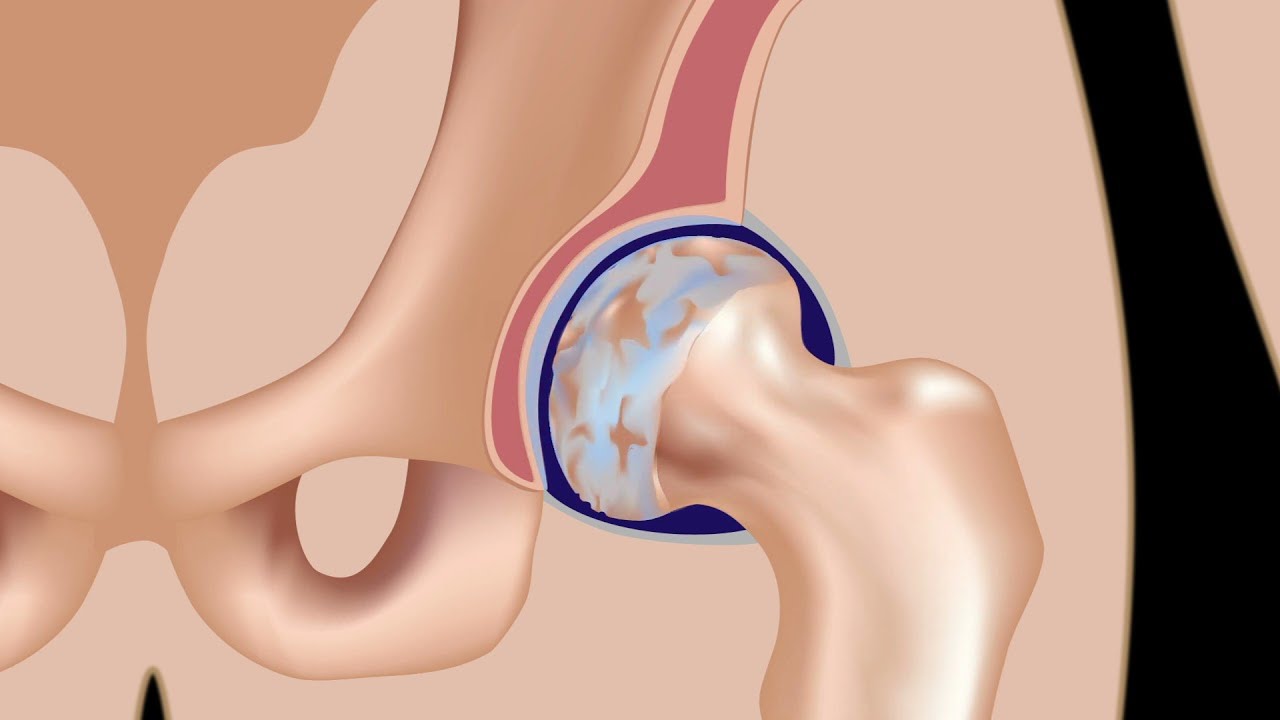The image is a detailed, cartoon-style anatomical rendering of the human hip joint, typically found in a medical textbook. It showcases the pelvic bones and the top portion of the femur where it forms the ball-and-socket joint. The hip joint's ball is highlighted within a dark blue circle, indicating cartilage, while the socket has a red hue. The illustration uses shades of light brown, white, and a hint of reddish-purple to depict the different bone structures and interstitial spaces. The background is black, contrasting with the monotone colors of the bones. There is also a detailed representation of the tailbone and parts of the pelvis, suggesting the image focuses on how these bones connect and function together.